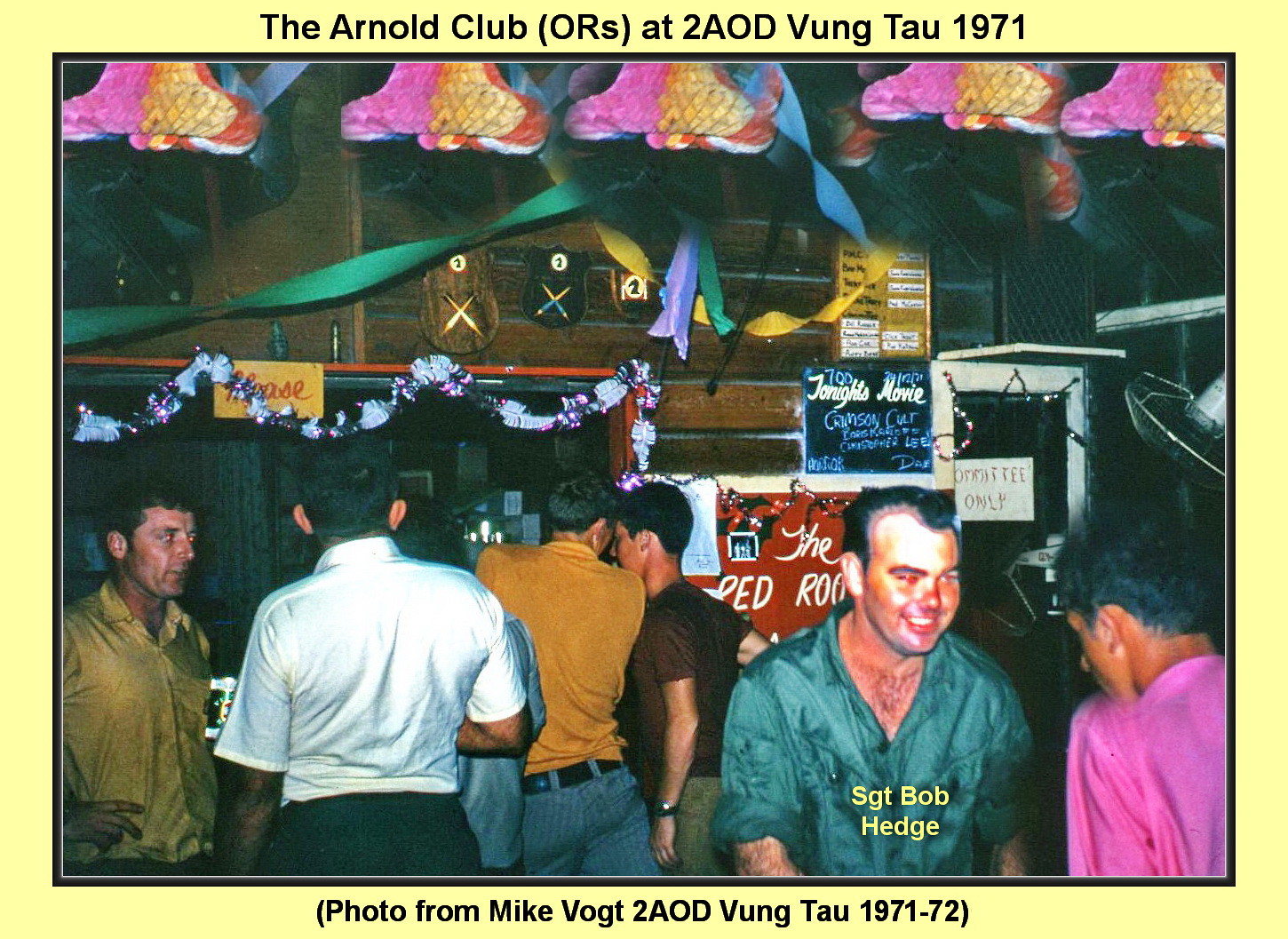The image is a color photograph taken inside a club called "The Arnold Club," also labeled O-R-S, located at 2 AOD Vung Tau in 1971, during the Vietnam War. The photograph is inset into a larger yellow background with a black headline at the top that reads "The Arnold Club" (O-R-S) and "at 2 AOD Vung Tau, 1971", and a caption at the bottom that states, "Photo from Mike Vogt, 2 AOD Vung Tau, 1971-72". In the foreground on the bottom right is a man in a teal shirt identified as Sergeant Bob Hedge, with his name superimposed in yellow font on his chest. The image captures a group of Caucasian men in their late 30s to early 40s socializing and facing each other inside a club, with some facing the camera and some facing away. The club has a festive atmosphere with paper crepe bells in pink, yellow, and blue, along with colorful streamers overhead. There are signs on the back wall, including movie signage for "Crimson Car", along with a few plaques, contributing to the party ambiance of the scene.